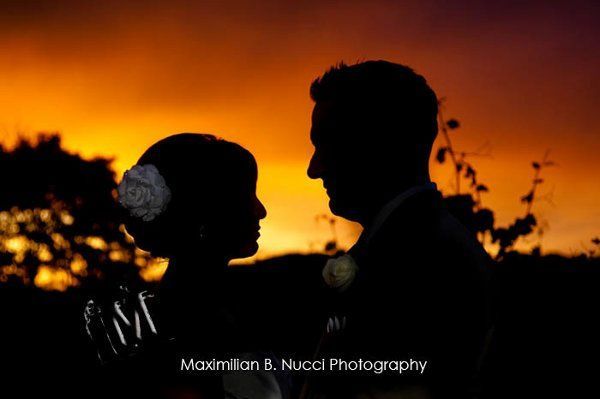The image captures a romantic silhouette of a man and a woman facing each other against an enchanting dusk sky. The background transitions from deep orange and brownish hues at the top to a lighter orangey-yellow near the horizon, suggestive of the last moments of sunset. To the left of the image, a tree stands as a dark silhouette with some grass or bushes edging the right side. The woman, positioned on the left, has a large white flower adorning her hair and appears to be wearing a white dress, while the man on the right wears a dark suit with a flower pinned to his left lapel. Both figures are backlit, highlighting their profiles in a tender moment. At the bottom of this rectangular, horizontal photo, the text "Maximilian B. Nucci Photography" is prominently displayed in white. The overall ambiance suggests a serene, possibly wedding-related scene captured in a beautifully blurred focus.